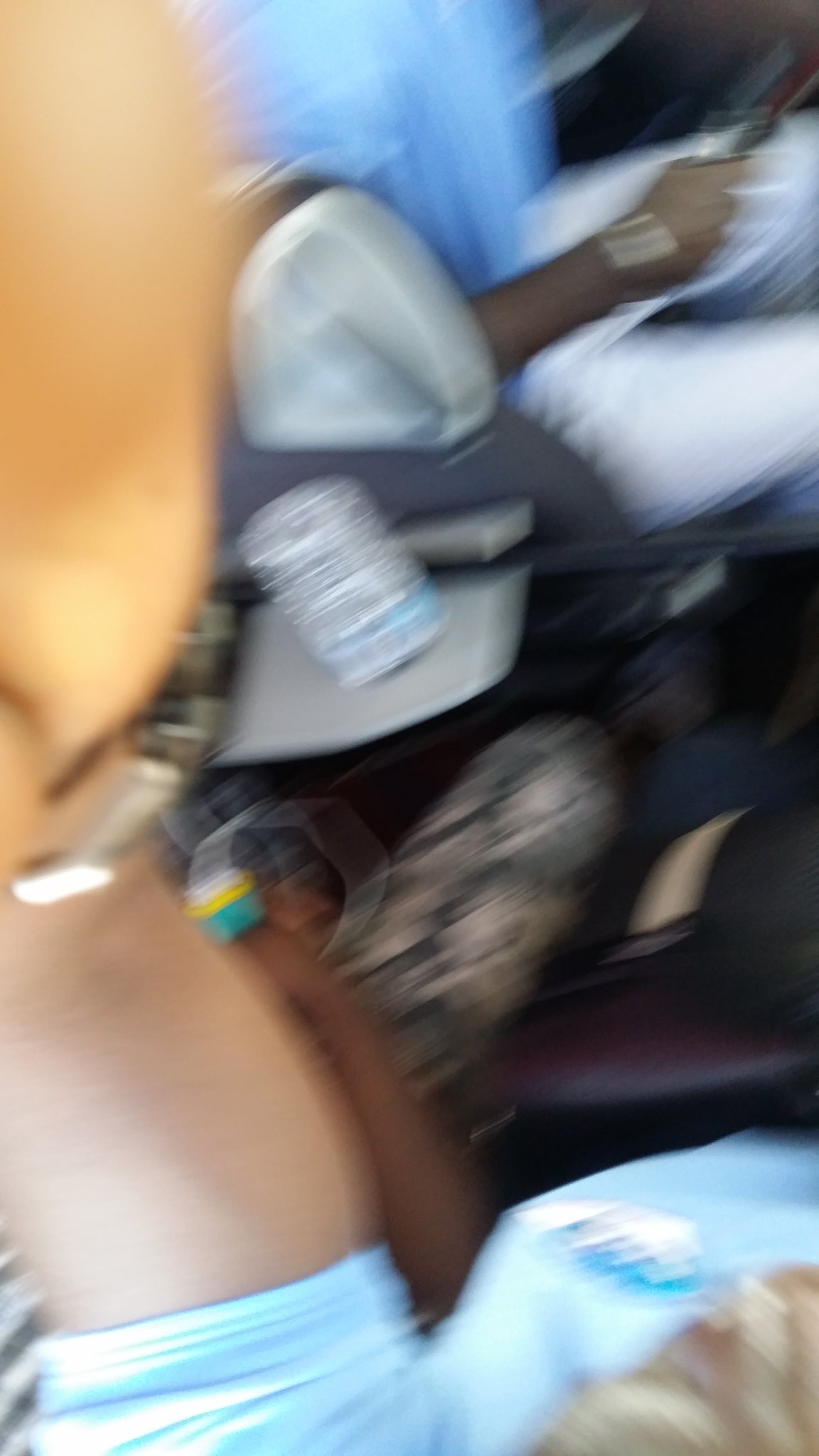This extremely blurry photograph, taken in a vertical orientation, captures a scene that appears to be in motion, making it difficult to determine the exact setting. In the foreground, from the perspective of the person taking the picture, we see a dark-skinned individual's leg, possibly wearing a light blue shirt. This individual is reaching out an arm towards the upper part of the image. The background features another person, likely an African-American man, wearing a light blue shirt with sleeves and white pants, seated in a gray chair. Various objects are scattered in the midsection of the image, including a white can with black lettering, a water bottle, and perhaps a small purse. The entire scene is very streaky with blue and white colors, contributing to the difficulty in identifying specific details. The gentleman in the background appears to be holding an object, possibly a remote control, and has something on his wrist, adding an additional layer of intrigue to this enigmatic and dynamic snapshot.